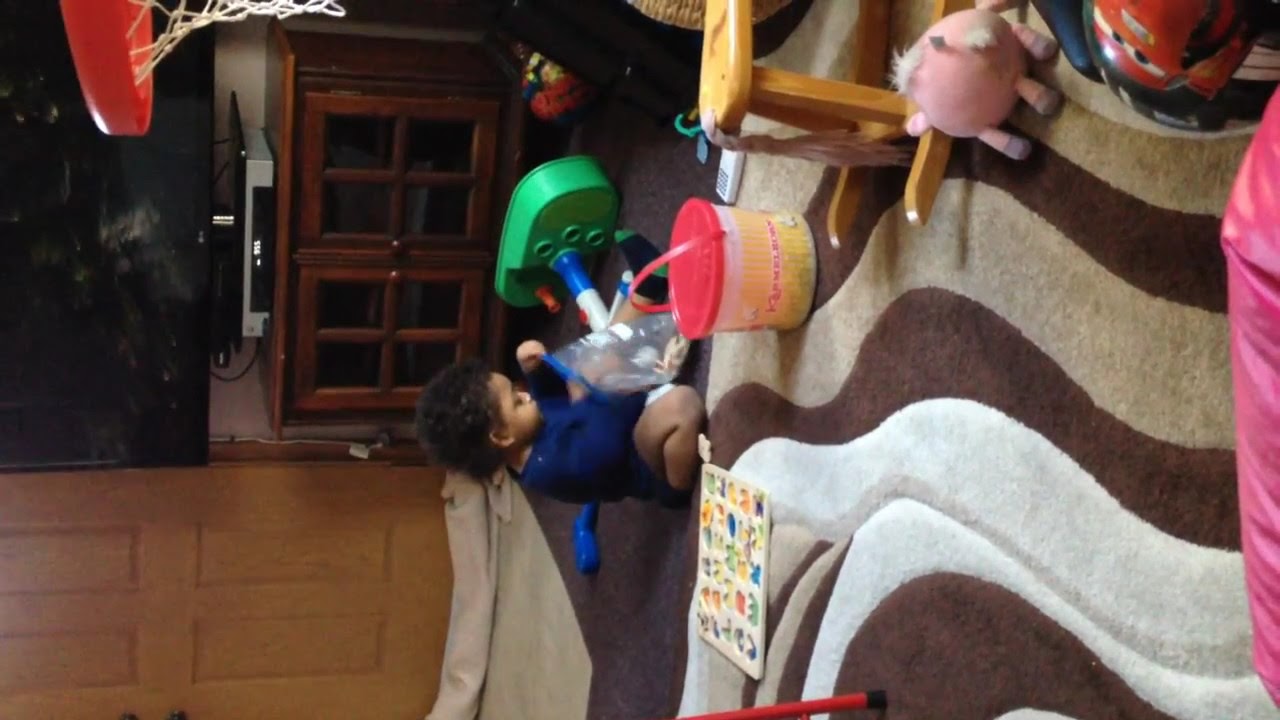The image, flipped 90 degrees counterclockwise, showcases a cozy living room scene centered around a small child. The child, likely around two years old, is light-skinned and wearing a blue onesie. Sitting on their knees, the child is engaged with a Ziploc bag, surrounded by an assortment of toys. The living room floor features a gray, brown, and white wavy-patterned rug that is partially covered with toys, including an Easter basket bucket with a pink lid, a red and yellow bucket, a pink stuffed animal, and a wooden ABC puzzle mat. Just behind the child, there is a wooden entertainment center with a large flat-screen TV on top. A small wooden rocking horse and a miniature basketball hoop add to the playful atmosphere. A door can be seen in the background, completing the detailed snapshot of this homey and vibrant living space.